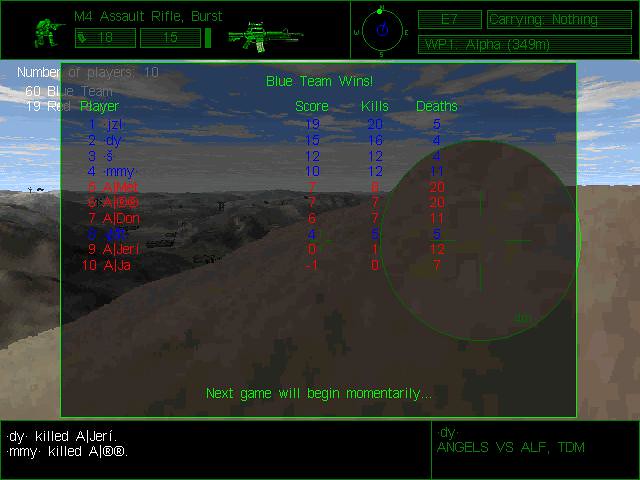The image appears to be a pixelated screenshot from an old-style shooter video game showing the end-of-game results. Dominating the screen is the announcement "Blue Team Wins," with player statistics listed below for ten participants, including scores, kills, and deaths. Players are identified by a mix of initials and names such as "Jerry" and "Don," with "ALJerry" notably in 9th place. Below the scoreboard, a ticker-like text provides real-time updates on in-game events, indicating actions like "dy killed a Jerry" and "MMY killed notes." The background features a prairie landscape with a blue sky, white clouds, and two brown mountains, which are simplistic and pixelated. On the top of the panel, "M4 Assault Rifle Burst" and radar graphics in neon green are visible, further confirming the shooter game genre. The screen also indicates the impending start of a new game with the message "Next game will begin momentarily."